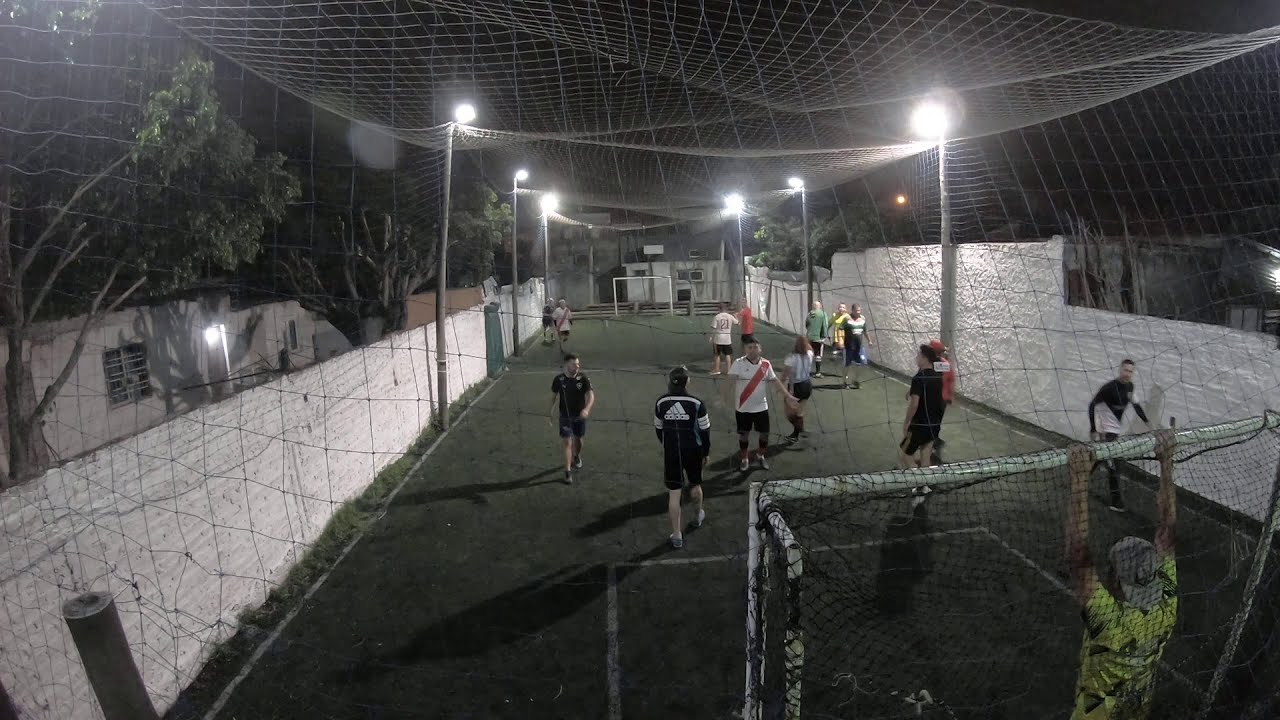The photograph captures a small, compressed soccer field set in an outdoor environment at night. The field, roughly 20 feet wide, is surrounded by netting on the sides and above to prevent the ball from flying out, with wooden fencing painted white along the perimeter. The netting is supported by tall wooden poles topped with streetlights that illuminate the scene. The setting appears to be a modest courtyard, possibly in an impoverished area, with clapboard or trailer-like homes and a few trees in the background. 

At the bottom right, a player in a black shirt is identified as the goalie, hanging onto the goal bar. The players on the field, possibly numbering around a dozen, range in age from children around 10 or 11 years old to adults, all dressed in mismatched jerseys and shirts, indicating an informal game rather than an organized match. The field is covered with artificial turf, and shadows are cast on the ground by the lights. In the distance, a second court is visible, also illuminated. The scene exudes a sense of community and casual play against a backdrop that hints at everyday resilience.